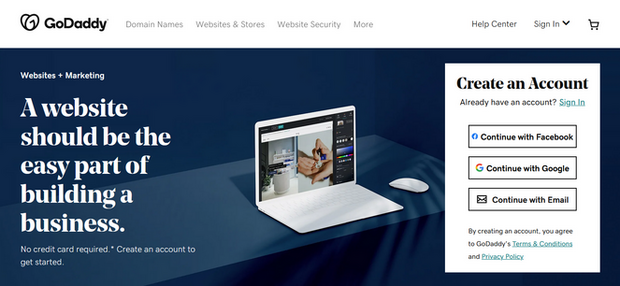This screenshot features the homepage of the GoDaddy website. In the upper left corner, the GoDaddy logo is displayed in bold text, accompanied by a heart-shaped emblem to its left. Directly to the right of the logo, there is a gray navigation menu listing options such as "Domain Names," "Websites & Stores," "Website Security," "More," "Help Center," and a "Sign In" button with a downward-pointing arrow. A shopping cart icon completes the top right section.

Below the navigation menu, a blue rectangular banner spans the width of the page, showcasing the slogan in white bold text: "A website should be the easy part of building a business." Beneath this, in smaller white text, the message continues: "No credit card required. Create an account to get started."

To the right side of the banner, a white laptop rests on a dark table, accompanied by a white mouse positioned to its right. Further to the right, a white call-to-action box invites users to "Create an Account." The box also provides options for existing users to "Sign In" and for new users to continue with Facebook, Google, or email.